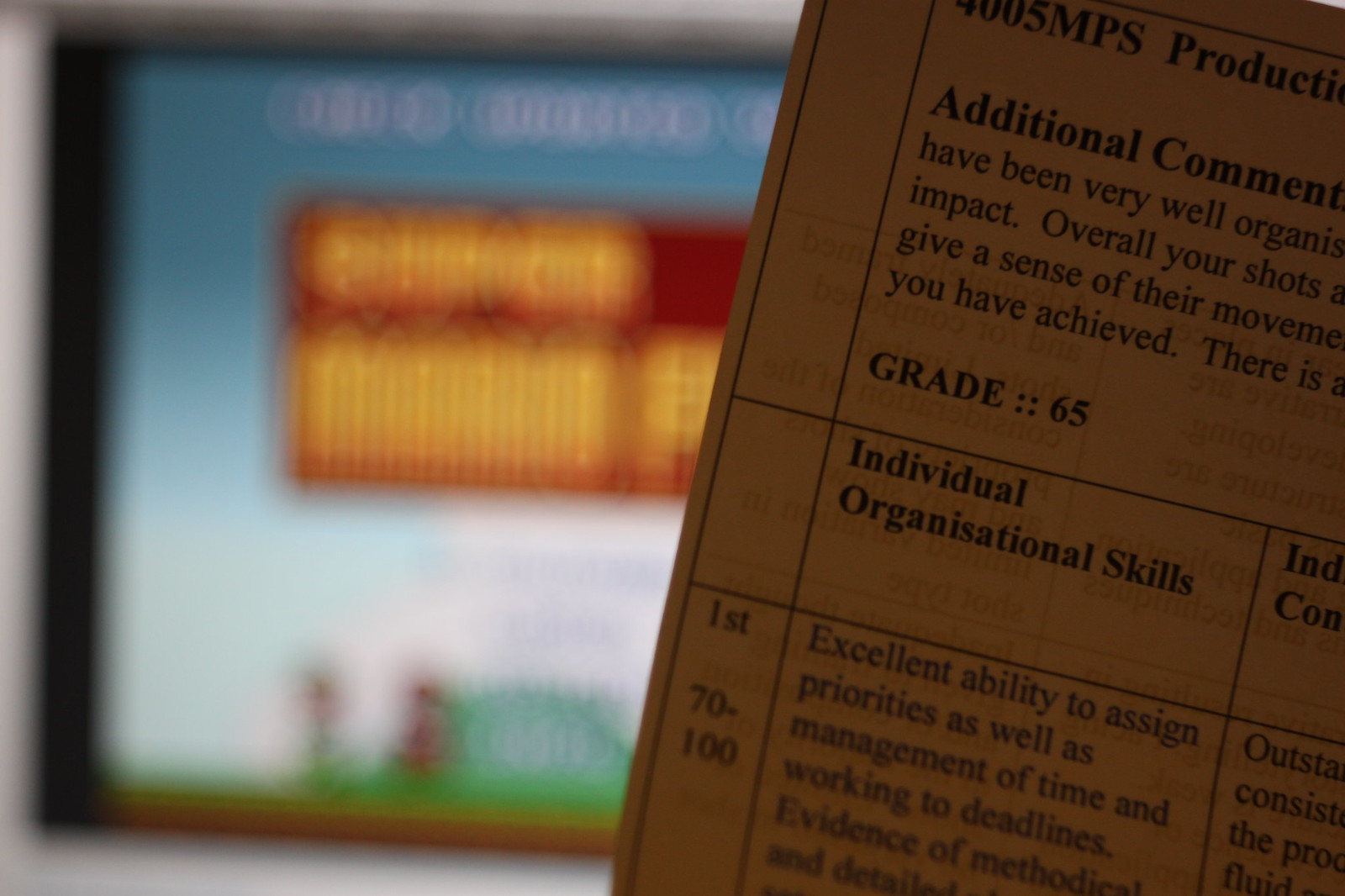The image captures a dark yellow-beige piece of paper on the right-hand side, resembling a report card or review document, typed in a standard font. This document is neatly organized into a grid format, featuring different categories and corresponding grades. The visible entries include "Additional Comments" with a descriptive paragraph below that mentions a grade of 65, focusing on qualities such as the organized impact of the individual’s work and their ability to convey movement through shots. Another visible category is "Individual Organizational Skills," highlighting excellent ability in prioritizing tasks, managing time, and meeting deadlines, with a grade range starting from 70-100. The left side of the image reveals a blurred TV screen displaying the title screen of the classic Super Mario Bros. video game, providing a nostalgic backdrop to the foregrounded document.